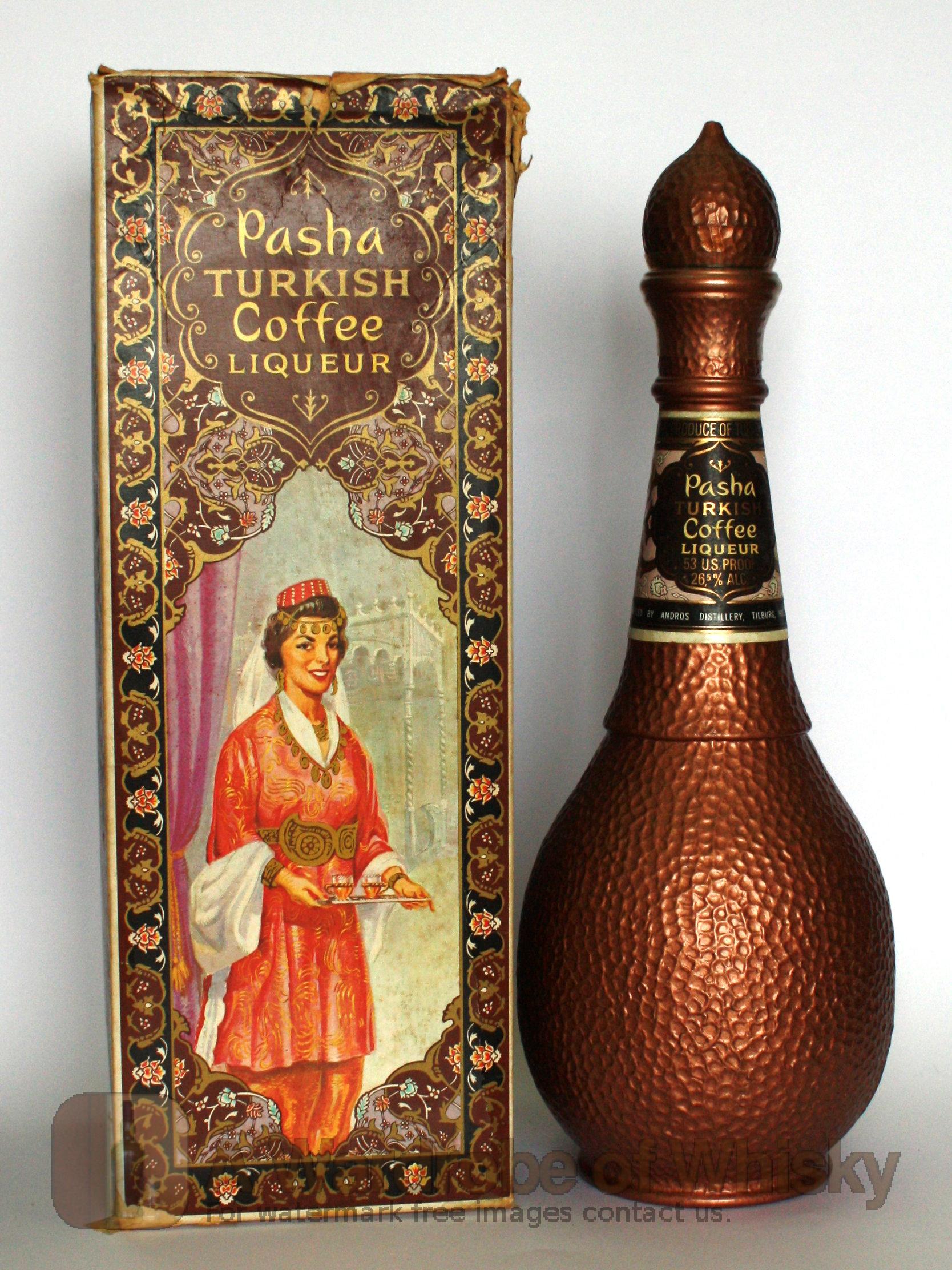The image showcases a refined and exotic bottle of Pasha Turkish Coffee Liqueur on the right side. The vial, appearing to be made from metal with a hammered texture, has a bronze hue, expanding from a circular base to a slender top. It bears a sophisticated black and gold label that reads "Pasha Turkish Coffee Liqueur," detailing its 26% alcohol content. Adjacent to the vial, on the left side of the image, is the packaging box, adorned with intricate, baroque-like decorations. The box prominently features the same "Pasha Turkish Coffee Liqueur" branding in elegant gold lettering. Below the text, there is an illustration of a woman dressed in expansive traditional Turkish attire complete with elaborate gold detailing and a fez hat. She is holding a tray with two cups of the liqueur, emphasizing the cultural essence and luxurious presentation of the product.